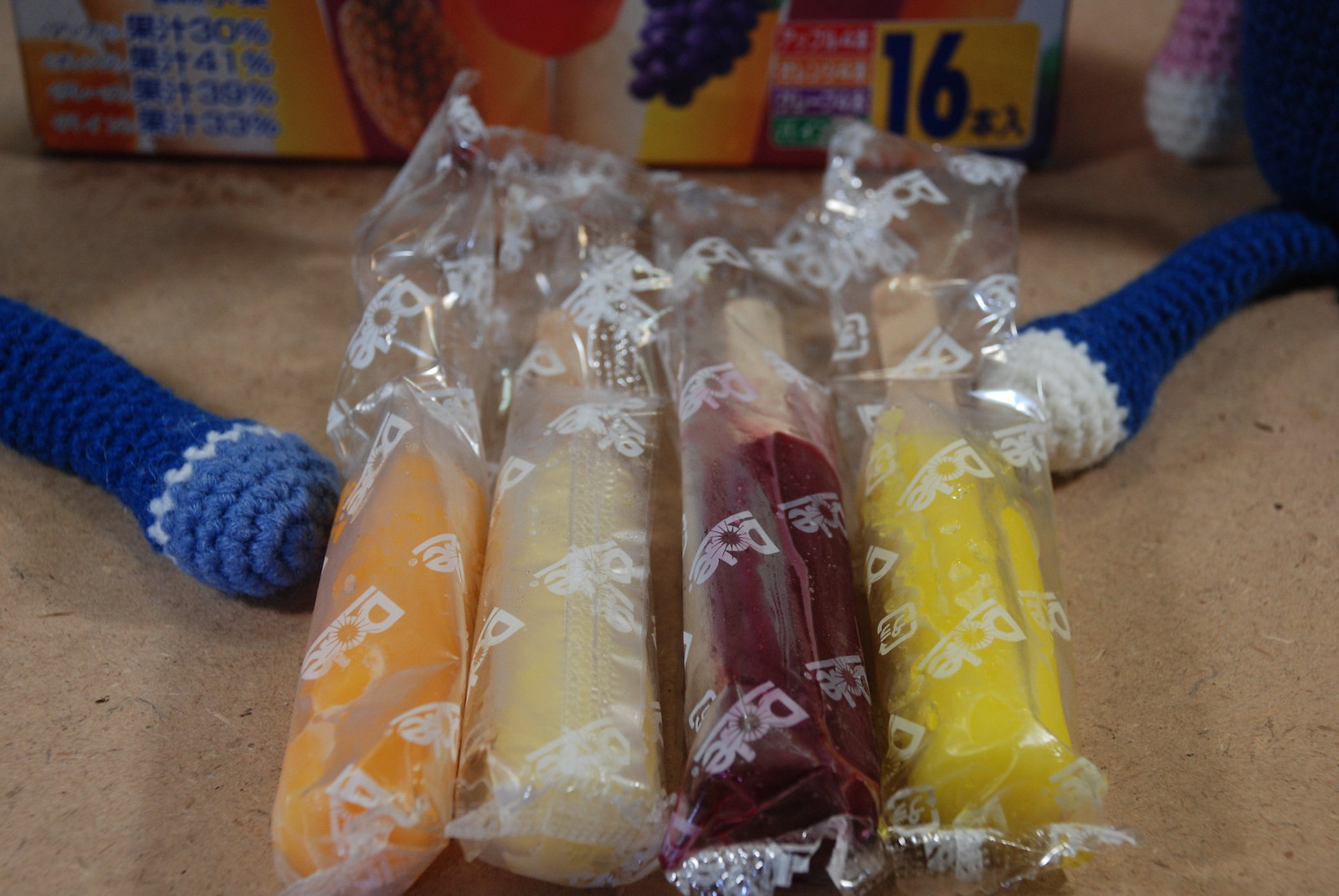This is a color photograph featuring four Dole fruit popsicles in their transparent cellophane wrappers, prominently displaying the Dole logo in white text. The popsicles, laid out in the center of the image, range in color from light orange, to pale yellow, dark reddish-purple, and bright yellow. The popsicles are all on sticks, pointed toward the top of the image, and rest on what appears to be a brown fiberboard or dirt-textured surface. Flanking the popsicles are two crocheted cylindrical pieces of fabric. In the background, the top of a colorful box, identified by Japanese text and the number 16, can be seen peeking out from the upper edge of the image.